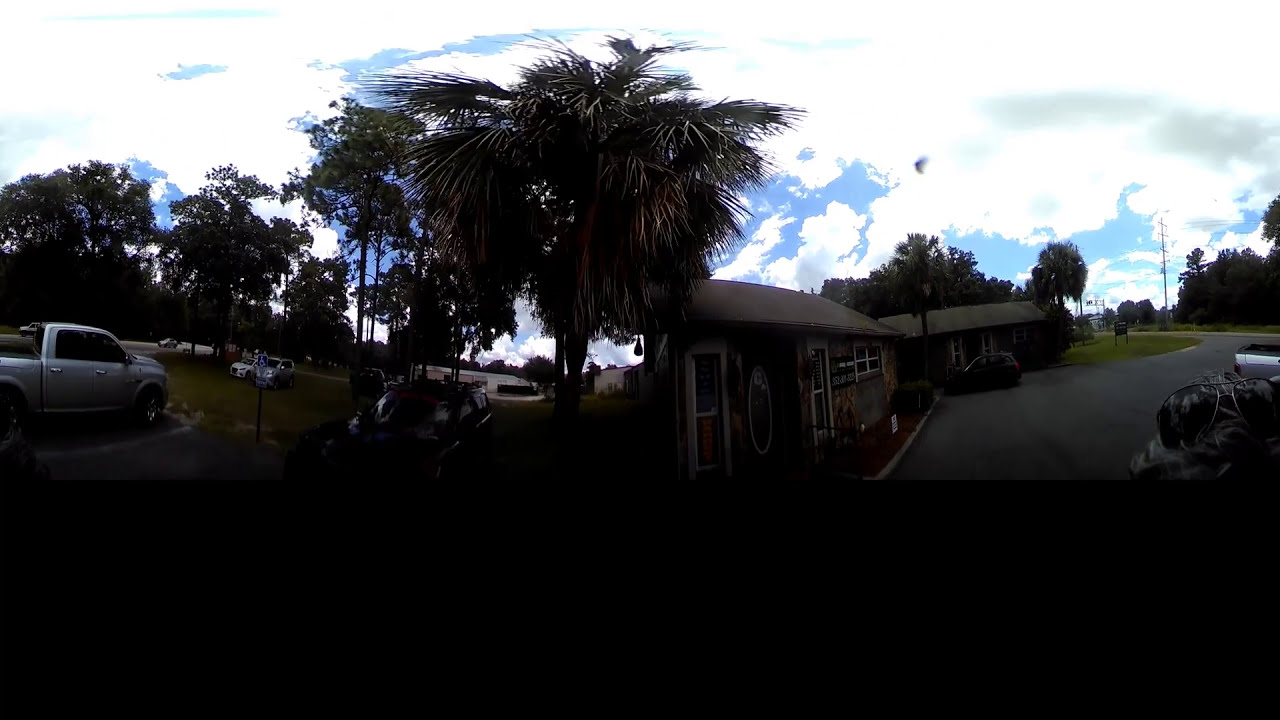In the rather dark image, there is a mix of houses and vehicles set against a cloudy sky with patches of blue. The main focus consists of two adjacent houses in the center. The house in the front features a distinctive oval-shaped window flanked by two additional windows. This house has a green exterior with white windows. A car is parked in front of the second house, which is partially obscured behind the first. 

The scene is densely populated with trees, which are visible in various positions across the image, including some far in the background. On the left-hand side, there is a white truck parked next to a disabled parking sign. A palm tree stands behind the house with the oval window, and to its left is a parked motorcycle, adjacent to a grassy area. Additional parked cars can be seen throughout the scene, suggesting this area might be a residential neighborhood, potentially with facilities for parking like a small lot. There also appears to be a road extending on the right side of the image. The mix of houses, vehicles, and various elements contributes to a slightly ambiguous setting, creating a snapshot of a densely utilized space.